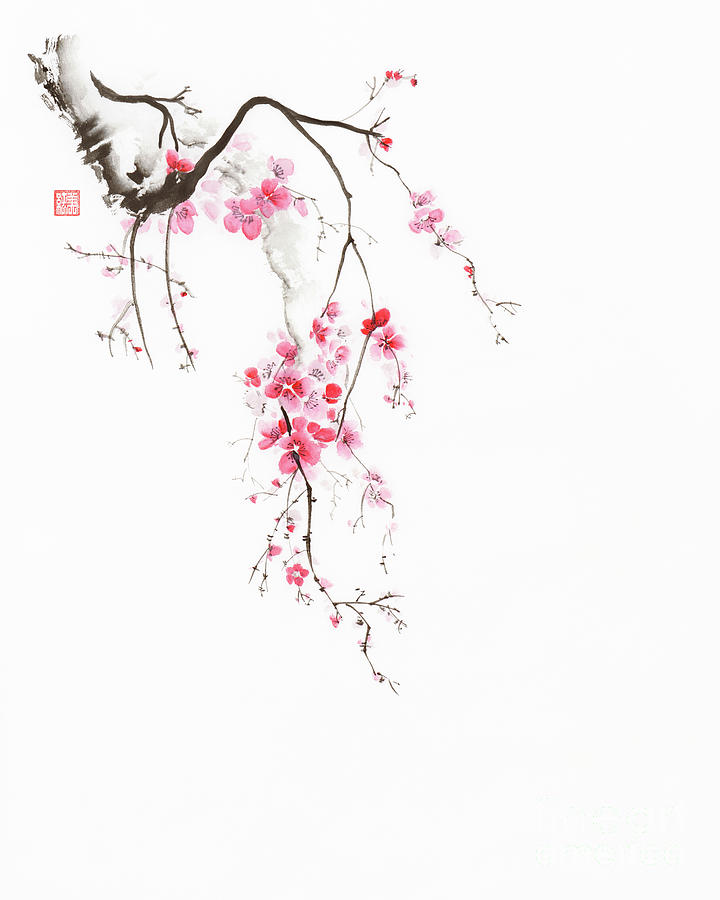This is a highly detailed, photorealistic painting set against a plain white backdrop, done in a classic Japanese style. The focal point of the image is a cherry blossom branch that extends from the top left corner, initially thick and shadowy, tapering into thinner branches. These thinner branches are adorned with an abundance of small, bright pink cherry blossom flowers, interspersed with occasional white blooms. The composition includes five or six branches, predominantly hanging low, with one or two branches extending higher. Additionally, there is a red signature square with intricate details on the left side, though the markings are too tiny to be decipherable. The overall effect is a stunning, almost photographic depiction of a cherry blossom branch, capturing both the elegance and delicate beauty of the flowers.